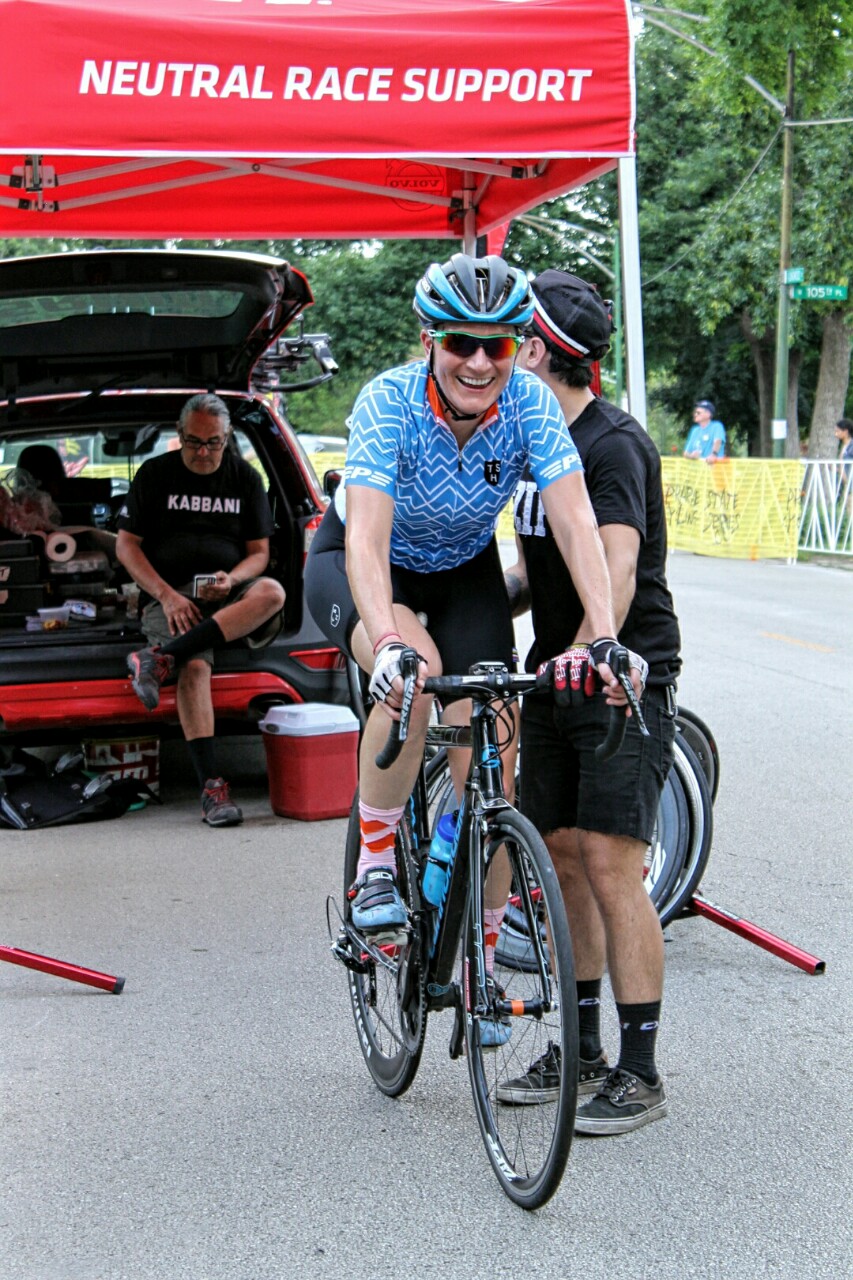In the photograph, there is a woman on a stationary bike, wearing a blue shirt with a white zigzag design, black shorts, and a black helmet with blue borders. She is also wearing glasses. To her right, a young man in a black shirt, black shorts, black socks, light gray shoes, and a black cap with red and white stripes is holding the bike steady. In the background, there is a red car with its trunk open, and an older man wearing a black shirt with the white text "Kabbani" on it is sitting on the edge of the trunk. A red cooler sits on the ground beside him. The scene takes place outside during the daytime under a tent that bears the text "Neutral Race Support," suggesting a race or cycling event.